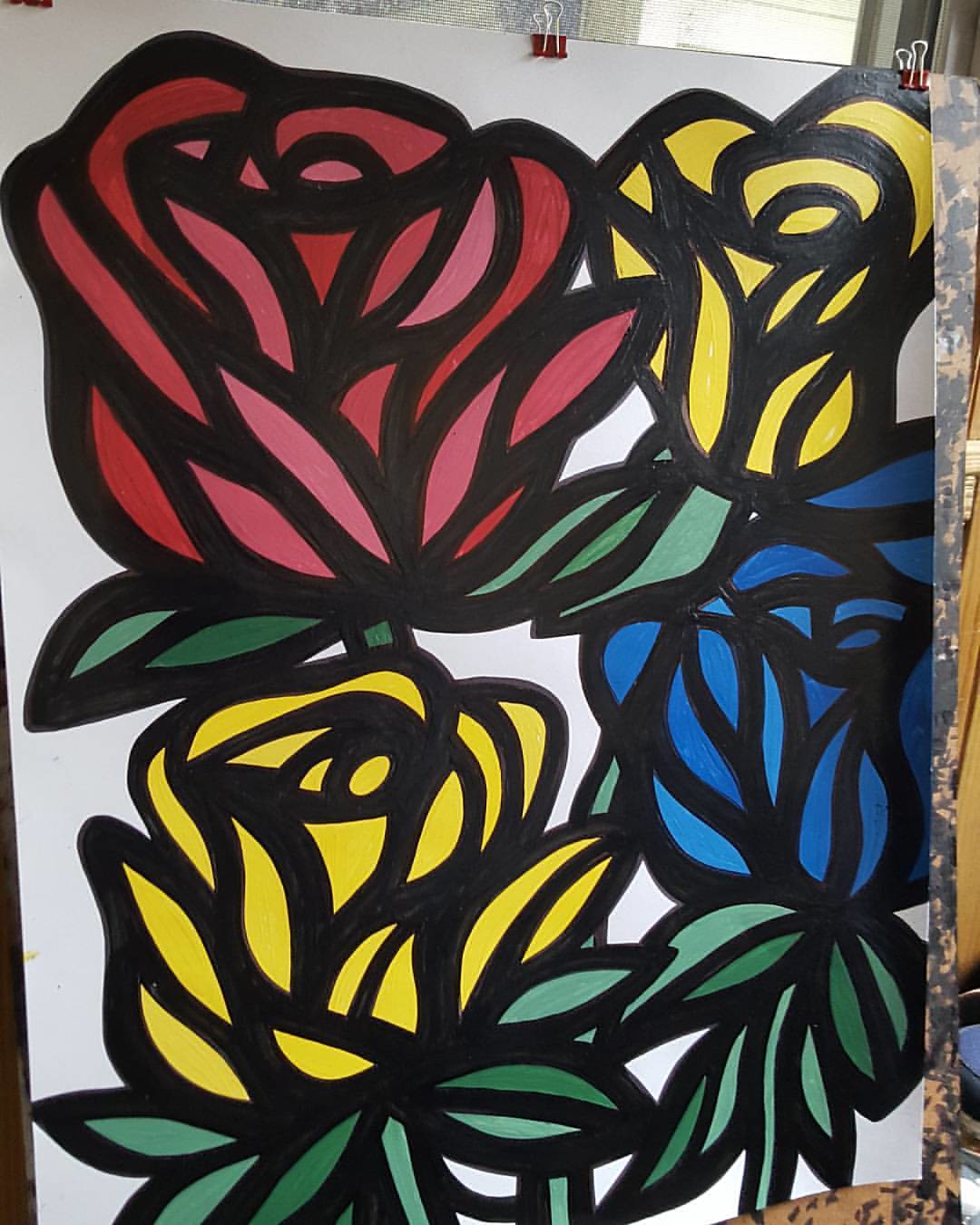This photograph features a large painting secured to a board with three red clips. The painting's background is predominantly white, while its subject matter consists of four vividly colored flowers arranged in a square formation—two flowers atop and two at the bottom. The flowers are colored red, yellow, yellow, and blue respectively, each featuring thick black outlines and complemented by green stems and leaves. The scene appears to be indoors, as suggested by the visible window and some indistinct furniture elements in the background.